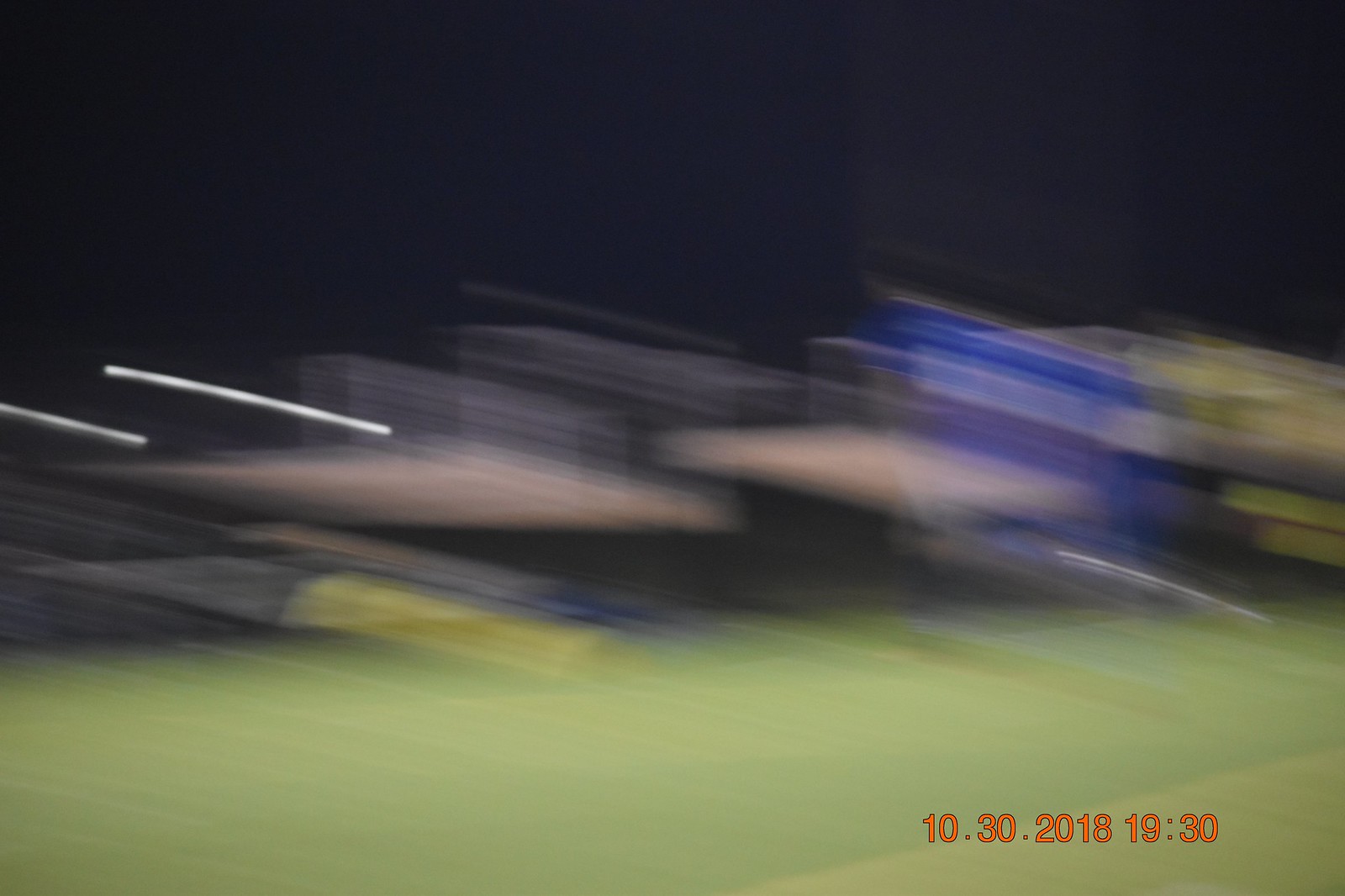Photograph dated October 30, 2018, timestamped 07:30 PM, taken on a digital camera as indicated by the orange date stamp in the bottom right corner. The image is blurry and appears to capture a scene in the evening or nighttime, possibly in a parking lot. The foreground shows a greenish-gray pavement, while the sky above is pitch black, suggesting darkness. Various indistinct light sources are visible, including flashes of blue, pink, and purple, which could be from signs or billboards. The overall atmosphere of the photograph is somewhat artisanal and abstract due to the blur and the mix of colors.